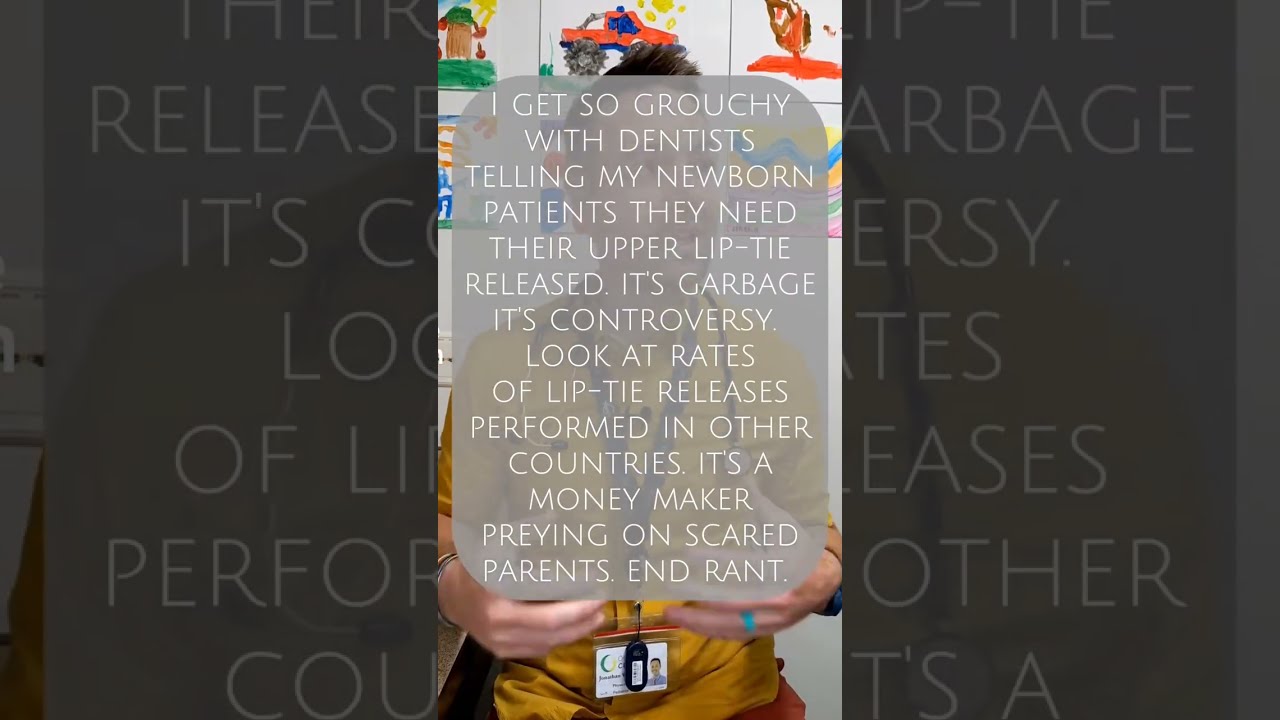The image features a central, vertically-oriented photograph of a dental worker in gold scrubs, identifiable by a lanyard with a photo ID around her neck, and brown hair. She stands in front of a wall adorned with children's colorful drawings—a gabled house, a red sports car, an all-terrain vehicle, and a plant on a red base. Superimposed on the photograph is a gray text cloud with white lettering that reads, "I get so grouchy with dentists telling my newborn patients they need their upper lip tie released. It's garbage. It's controversy. Look at the rates of lip-tie releases performed in other countries. It's a moneymaker preying on scared parents. End rant." The left and right sides of the image reproduce parts of this text in black and white close-ups, subtitled "Release. It's C-L-O-O-F-L-I-P-E-R-F-O-R-C-O" on the left and "Garbage or G-E-R-S-Y-T-E-S-E-A-S-E-S-Other-T-S-A" on the right. The entire composition presents a blend of graphic elements and photography, with the central photo in a portrait orientation highlighted against a darkened, horizontally-oriented, enlarged backdrop.